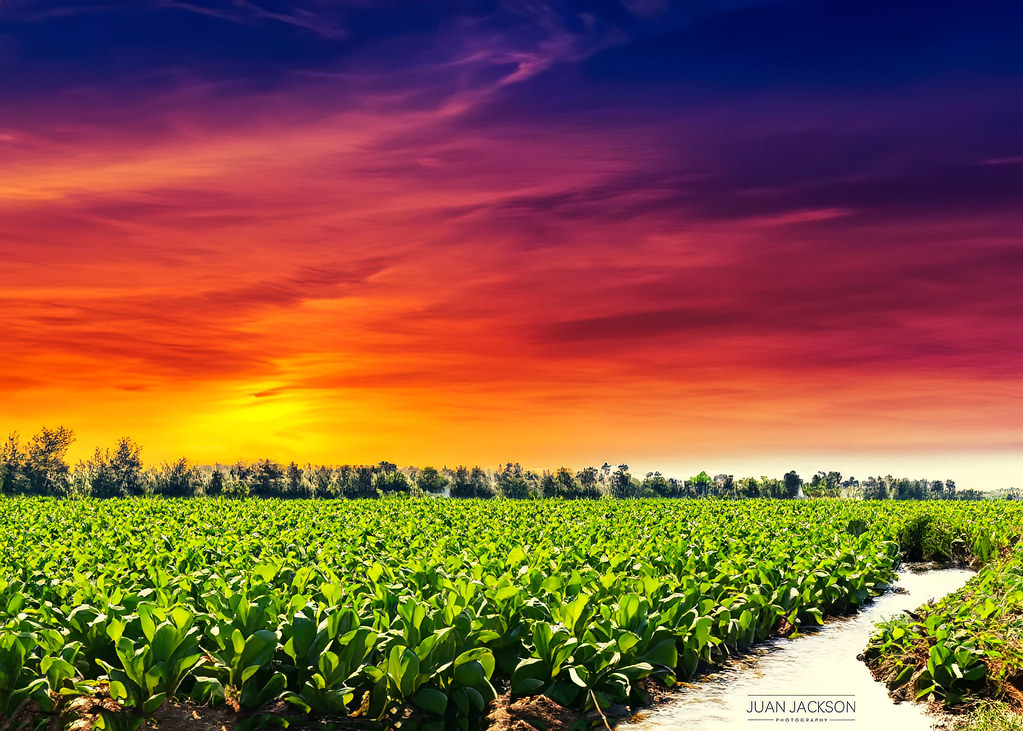A breathtaking landscape photograph by Juan Jackson captures a serene sunset on the horizon, casting a warm spectrum of yellow, orange, magenta, and deep reds across the sky, blending into the encroaching night. The sky's vibrant hues transition smoothly, painting the clouds in shades of orange, purple, and dark red. Below this dazzling display, a tree line of lush, green trees stands silhouetted against the colorful backdrop. The foreground features a thriving bed of verdant crops or plants, stretching out about three feet tall, their rich green tones contrasting beautifully against the brilliant sky. A charming gravel path winds gently through the greenery, creating a scenic route that draws the viewer's eye deeper into the photograph, reflecting the tranquil harmony of nature.